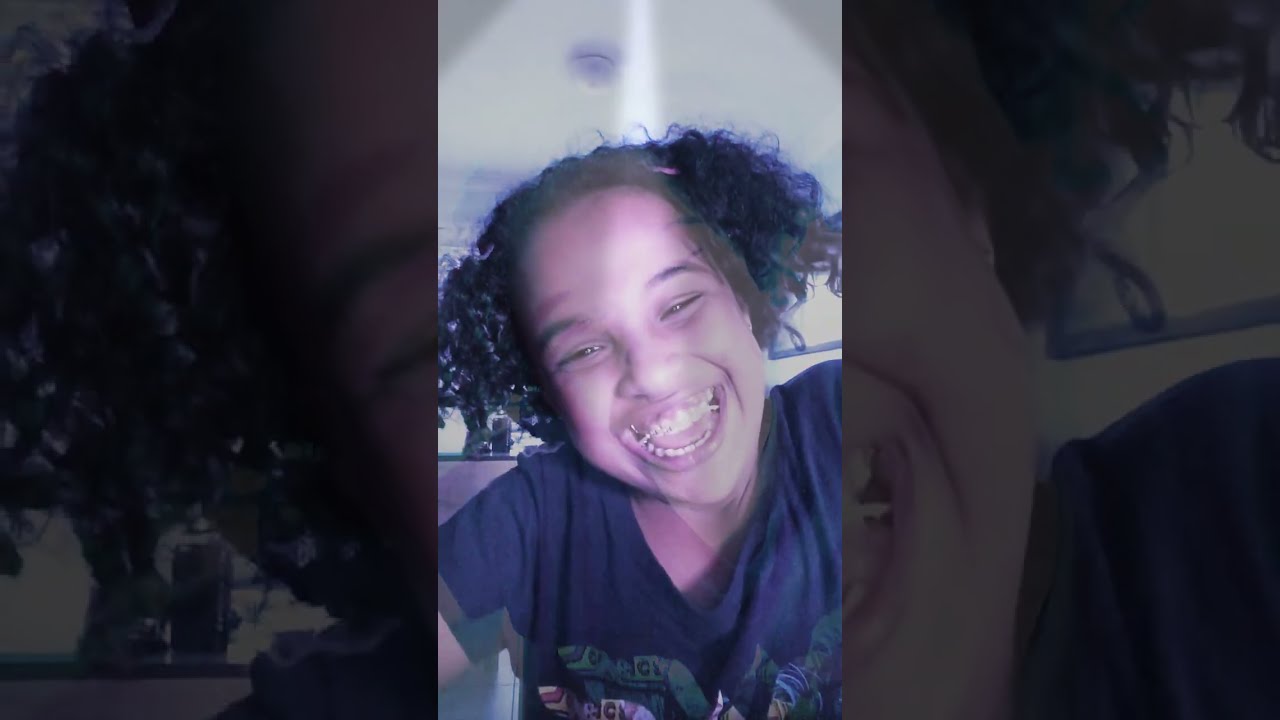The image features a light-skinned black child with tanned skin. She has a mouth wide open in a happy, laughing smile, showcasing her braces with little bands connecting the top and bottom jaws. Her short curly black hair is styled in pigtails. She is wearing a black t-shirt. The photograph has a white ceiling in the background with light streaming down onto her face, although the ceiling light itself appears to be turned off. Notably, the child's image is repeated and enlarged, framing the central picture with split faces on the left and right sides, merging into an artistic, mirrored effect. The photo is brightly illuminated by natural light, enhancing her joyful expression and clear details.